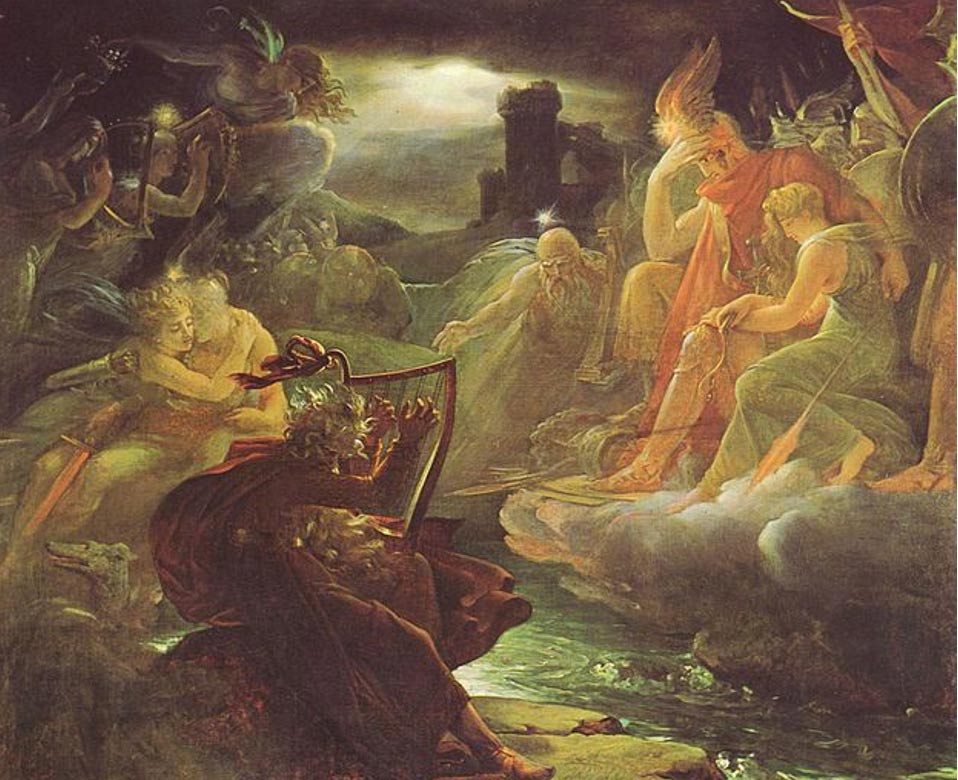The painting is an old, dramatized artwork reminiscent of Roman or Greek styles, possibly created centuries ago. It features a dramatic scene set amidst clouds under a stormy, dark sky with shades of gray and dark blue, and a bright light peeking through. Central to the piece is a distant, ethereal castle with numerous angelic figures spreading across the composition. On the left, angels with harps appear both seated and embracing. On the right-hand side, other angels are depicted armed with weapons such as spears, swords, and shields. Prominently, there is a figure in a red robe and a gold helmet adorned with wings, standing on a cloud with his arm around a woman in a green dress. To their right, partial views of more figures are visible, showing only their limbs. An old man with a flowing white beard stands centrally, his outstretched hand reaching towards a figure in a red cloak who faces away from the viewer, gesturing back towards the old man. The colors appear faded, giving the image a timeworn, museum-worthy quality.